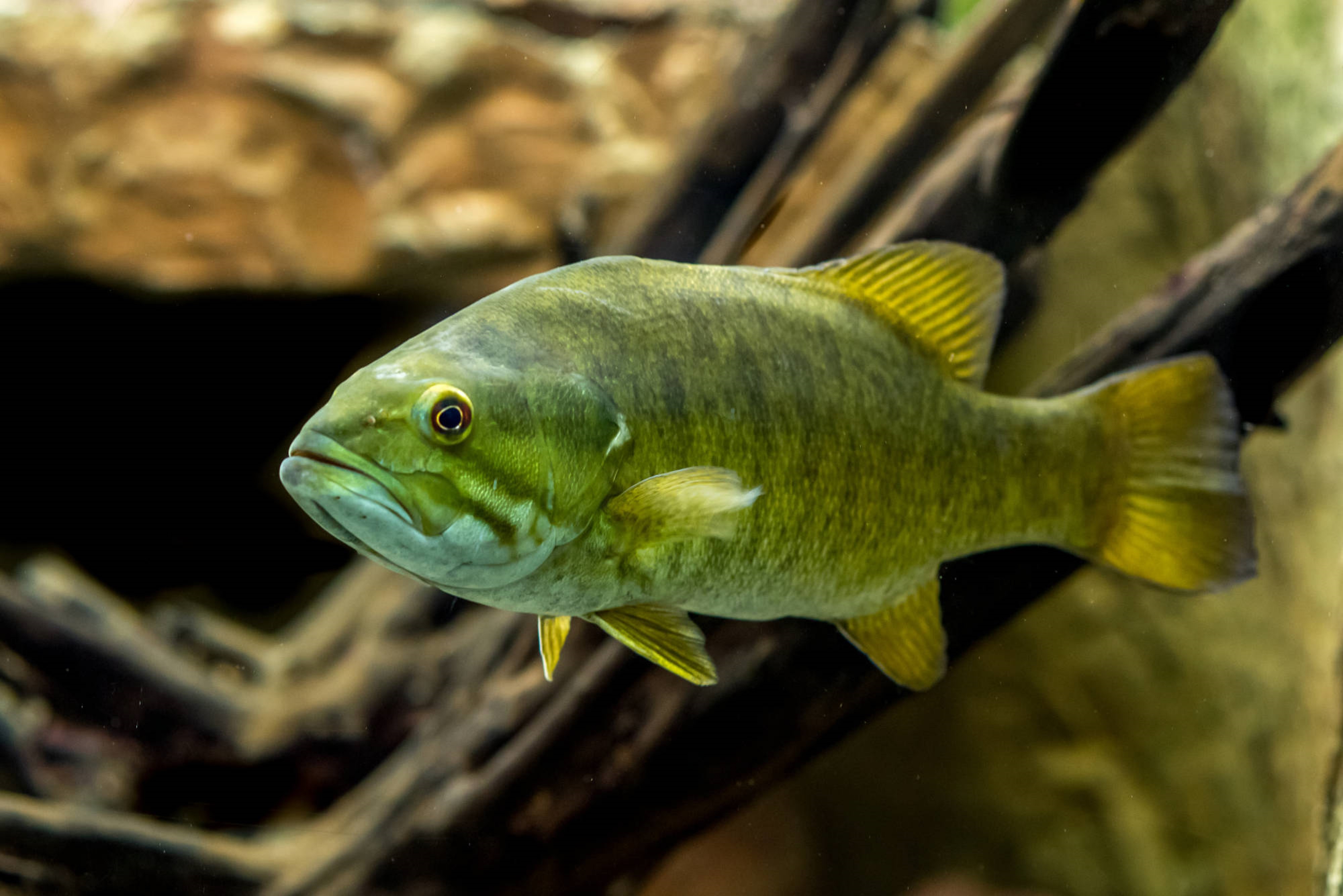The image features a single greenish fish prominently in the center, occupying about 60% of the frame and presented in a side profile with its eye looking straight at the camera. The fish's scales display various shades of green, and its fins glow with a greenish-gold or yellowish hue due to the light shining through. The eye is quite detailed, showing a perfect black circle surrounded by a thin yellow circumference. The background is a blurry bokeh mix of browns, blacks, and greens, suggesting a naturally murky aquatic habitat. The fish has distinct anatomical features including an upper fin, a tail fin, a bottom fin, and two front steering fins, along with gills or flappers on its body. Overall, the fish's vivid green coloration with hints of blue and yellow makes it the focal point of this detailed and serene underwater scene.